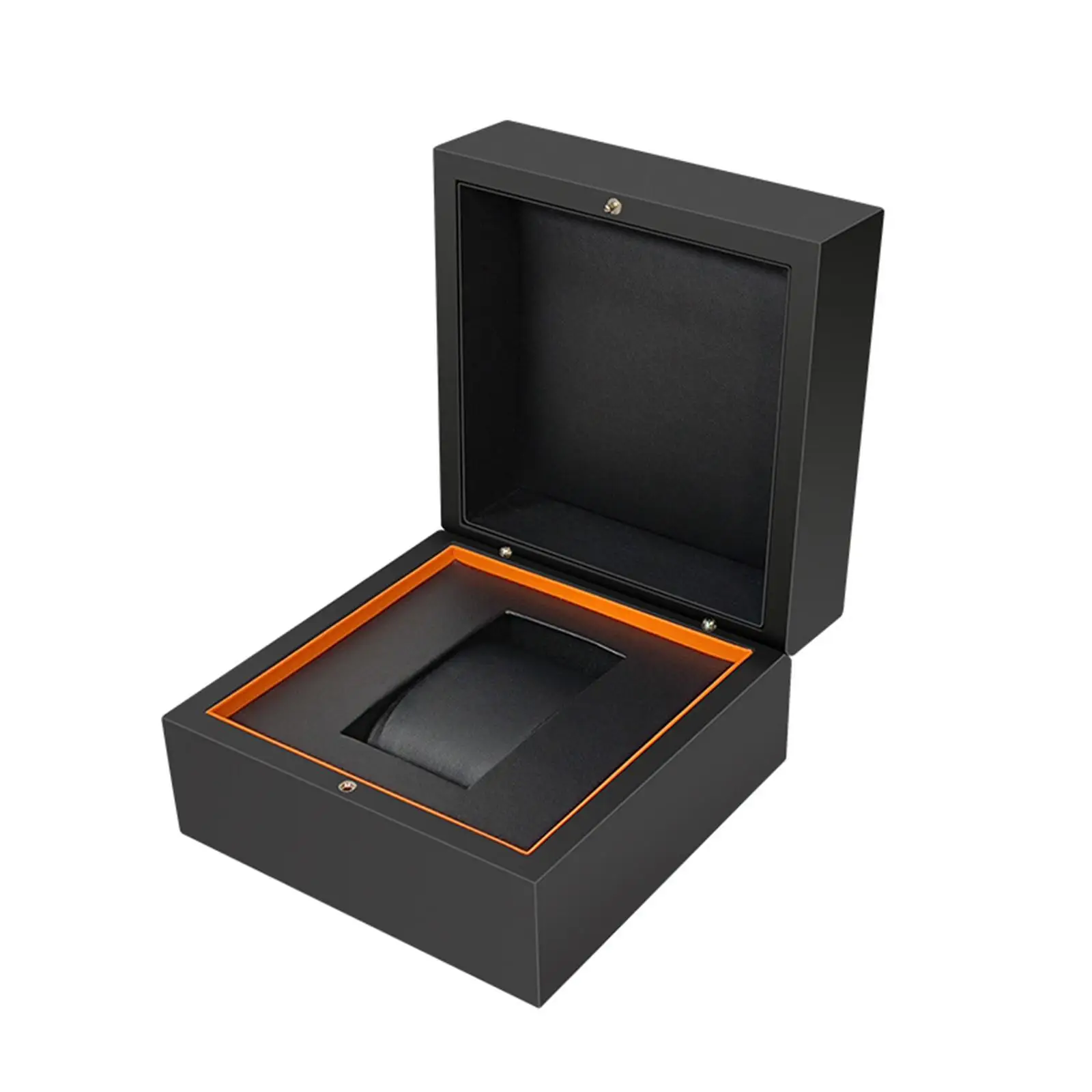The image depicts a detailed view of an open, elegant black box. The exterior and interior surfaces of the box are matte black, presenting a sleek, modern look. A distinct orange rim decorates the inside bottom half of the box, adding a striking contrast to its predominantly black finish. The box features a rectangular cutout in the middle, lined with cushion-like material, designed to securely hold an item, possibly a ring, watch, or tie. Additionally, the box includes a sophisticated locking mechanism with a hole and a corresponding protrusion that allows it to snap shut securely. The background of the image is completely white, drawing full attention to the open box and its intricate details.